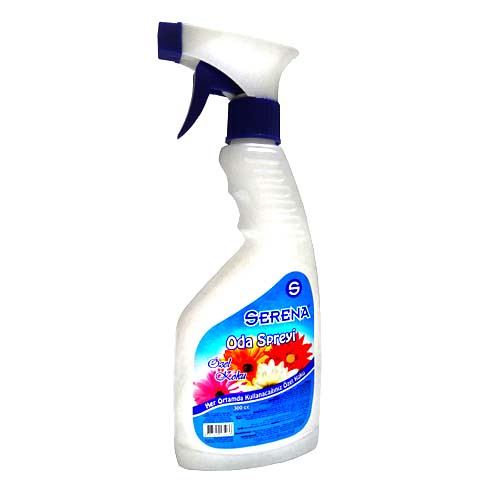This image features a white spray bottle accented with a dark blue cap, nozzle, and adjustable spray trigger. The bottle is set against a transparent background, highlighted by subtle shadows that delineate its contours. It prominently displays a blue label adorned with floral imagery—pink, orange, yellow, and white flowers—that enhance its appeal. Centered on the label is a notable white letter 'S' within a blue circle, accompanied by the brand name 'Serena' in bold blue text with a white outline. Below this, the label reads "ODA Spray," stylized as "O-D-A S-P-R-E-Y-I," indicating a probable non-English origin. Additional text beneath the flowers appears in cursive but is partially illegible. The lower part of the label contains further information, including instructions and a white barcode with black lines, all set against a continuation of the blue background with darker blue text.